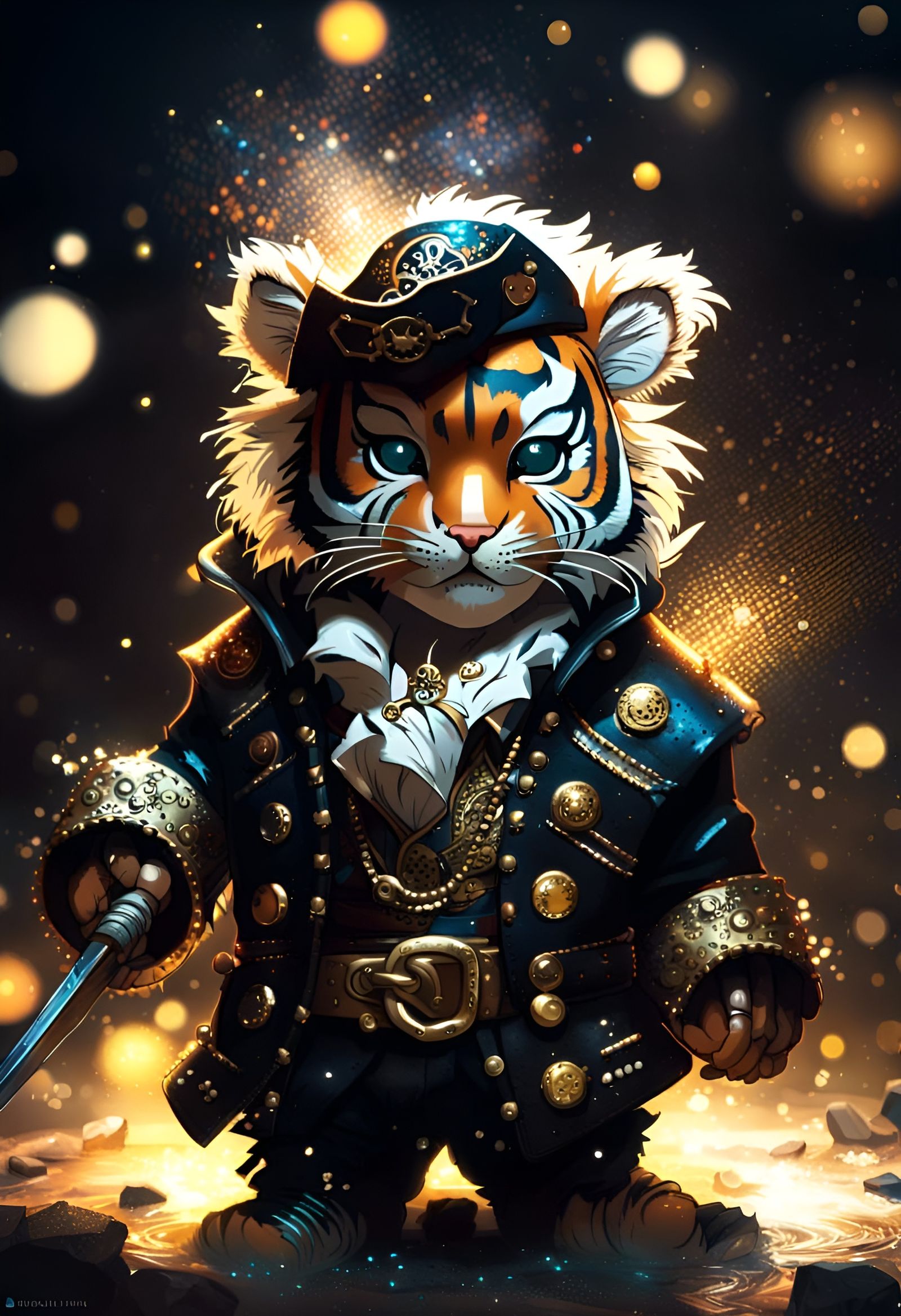The image is a detailed digital print of an anthropomorphic tiger dressed in an elaborate pirate outfit. The background features a dark sky illuminated by colorful lights resembling planets or confetti, creating a dramatic and festive atmosphere. The tiger, standing upright on its hind legs, has striking orange fur with black stripes and white accents on its face, including visible whiskers and a pink nose. Its black eyes are focused forward, adding intensity to its expression.

The tiger's attire is rich in detail, consisting of a dark blue pirate jacket adorned with gold buttons, embellishments, and metallic-looking cuffs at the sleeves. A matching dark blue pirate hat with gold and black details sits atop its head, with tiger ears peeking from underneath. A brown belt with a gold buckle cinches the tiger's waist, possibly complemented by a gold necklace and additional gold embellishments on a white shirt collar beneath the jacket. The tiger's feet are orange with black stripes, and it's unclear if they are bare or shod as they appear. 

In its right hand, which seems to blend characteristics of both paws and hands, the tiger wields a sword pointed forward toward the viewer. The scene is further brought to life by the reflection of light in a puddle at the tiger's feet, adding to the vivid, immersive quality of the artwork.